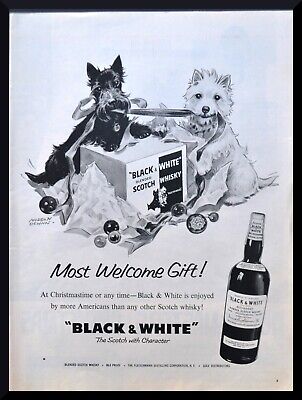This is a vertical black and white advertisement with a thin, solid black border. The upper two-thirds feature a white background with a detailed drawing of two dogs, a black Scottish Terrier on the left and a white dog on the right, both tugging on a black ribbon held in their mouths. In front of the dogs is a partially unwrapped white box with black writing on one side that reads "Black Scotch" and black coloring with white writing on the other side that says "White Whiskey." The scene is festive with black and silver ornaments and scattered wrapping paper, suggesting a Christmas gift. Below the illustration, the lower third of the ad is filled with black text that states, "Most Welcome Gift. Most Welcome Gift at Christmastime or any time. Black and White is enjoyed by more Americans than any other Scotch whiskey." Beside the text, on the bottom right, there's an image of a black bottle with a white label that says "Black and White." The tagline at the end reads, "Black and White in black letters, the Scotch with character."